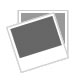This detailed watercolor painting, likely hand-drawn, captures a dramatic maritime scene set in what appears to be the 1700s or perhaps spanning centuries. Dominating the painting is a grand ship with three towering masts, proudly featuring an American flag on its left side along with another unclear flag at the top. The vessel battles choppy, cresting blue waves flecked with white foam, suggesting the onset of a storm. Surrounding the ship are approximately a dozen white seagulls, which, coupled with the foamy waters, imply proximity to the shore. The sky above blends hues of white and red, possibly hinting at a sunset, contributing to the painting's dynamic and somewhat tumultuous atmosphere. On the lower right side of the composition, a smaller vessel is also visible amidst the ocean swells. The intricate details, from the rigging of the ship to the bustling seagulls and the colorful sky, come together to create a vivid and evocative maritime scene.